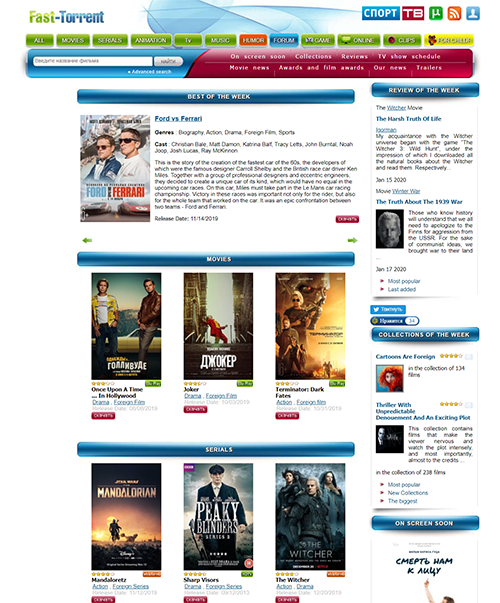Here's a detailed and cleaned-up caption for the described image:

---

The image is a screenshot from the FastTorrent website. In the top left corner, the FastTorrent logo is prominently displayed. On the upper right side, there is a blue button labeled "CNOPT," accompanied by a red box containing "TB" and a green box with the letter "U," likely indicating uTorrent. To the left of these elements, there is an icon resembling the RSS feed symbol, similar to Reddit's emblem, followed by a user profile square.

Beneath this top section, there is a horizontal menu featuring buttons that seem to represent various categories, mainly focused on movies and animation. Directly below this menu, a search bar is positioned towards the left side of the screen. The search bar turns red as it extends towards the right, indicating additional menu options.

The main body of the website is divided into three distinct horizontal sections in the center and a vertical section on the right. In the central area, one section is labeled "Best of the Week," another is titled "Movies," and the third is marked "Serials." The vertical section on the right provides supplementary content or features.

---

This version provides a structured and detailed description, making it easier for the reader to visualize the website layout.